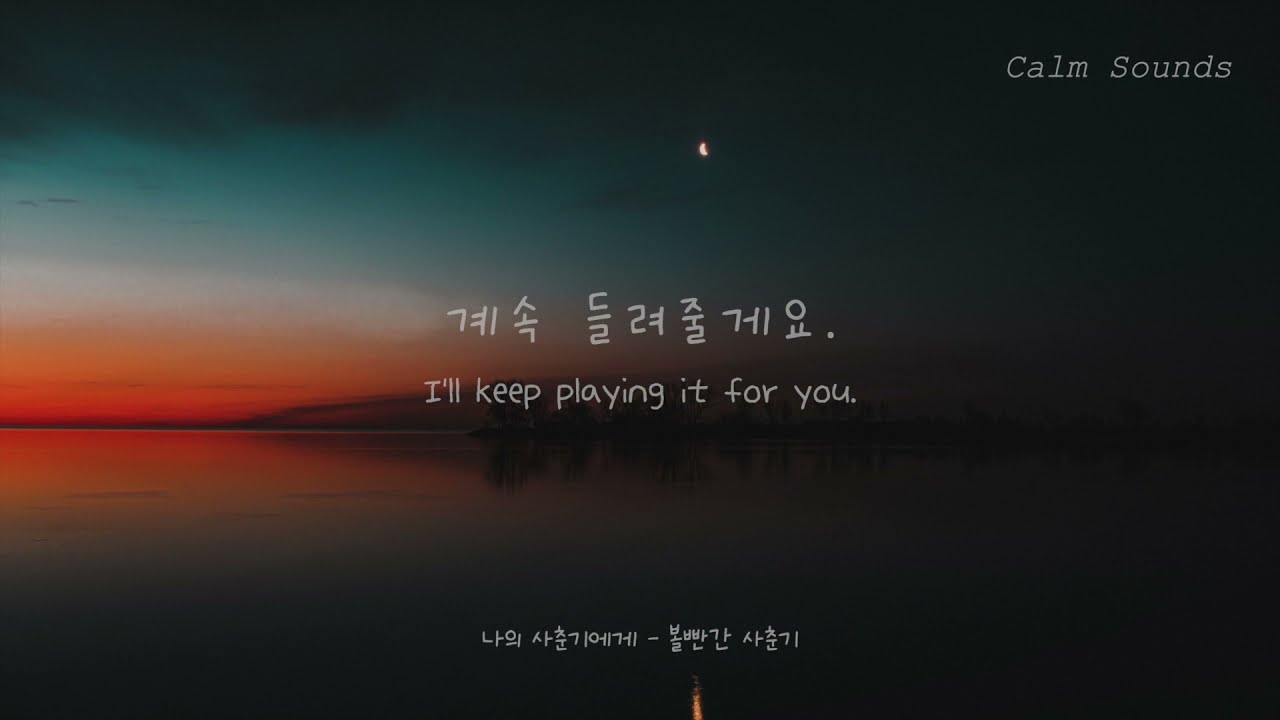The image depicts a serene evening or sunset scene, where the dark, tranquil waters of an ocean or lake reflect the vibrant hues of the setting sun. The sky, predominantly dark aqua, transitions from deep midnight green and black on the right to vivid reds, oranges, and yellows on the left, casting a rainbow of colors across the horizon. The upper right corner of the image features the text "CALM SOUNDS" in white, while the middle left side displays the phrase "I'll keep playing it for you." Above and below the image, there are foreign characters resembling Japanese or a Southeast Asian script, suggesting it might be a screen capture from a lyric video or promotional content. The image is shrouded in a dark border, adding to its peaceful and contemplative ambiance.